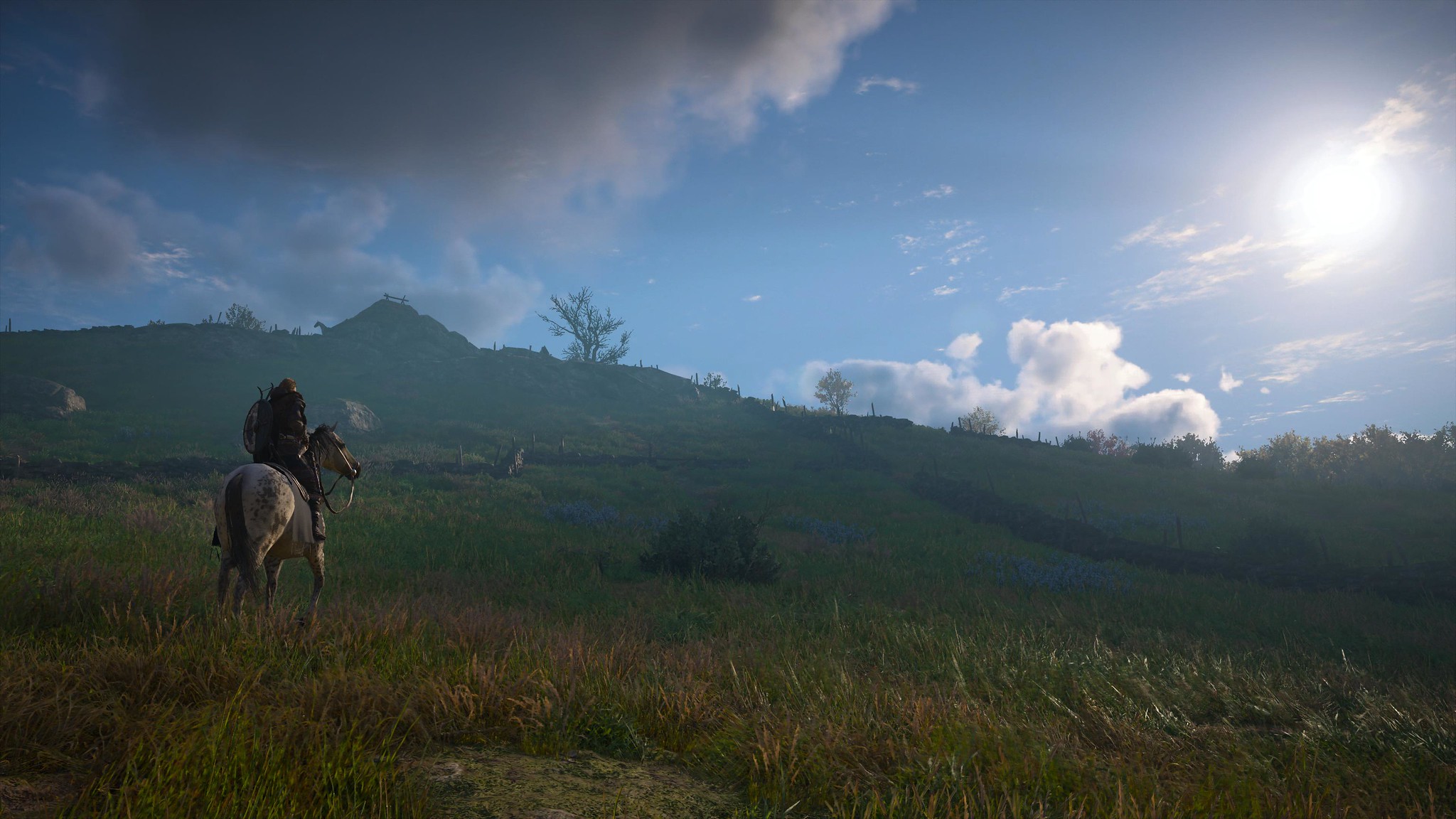The image resembles a highly realistic digital render, akin to a screen capture from a video game such as Red Dead Redemption, The Witcher, or Skyrim. It portrays a white horse with gray speckles, possibly an Appaloosa, ridden by an individual clad in detailed armor-like gear in blacks and browns. The horse and rider, though digital, appear strikingly lifelike. They stand in the foreground of a lush, rolling landscape comprising various patches of grass—brown, barren patches intermingled with long, green stretches. The scene's background reveals more green hills, a dirt patch left of center, and a ridgeline dotted with trees and possibly a barn or house, partly obscured by a silhouetted horse. Natural barriers, like rock or hedge lines, divide the fields. The lighting suggests the sun is positioned in the upper right, about an hour before sunset, casting a warm glow over the scenery. The sky is a remarkable blue, with fluffy white clouds underneath a bright sun. In contrast, darker storm clouds loom in the upper left, hinting at impending rain.